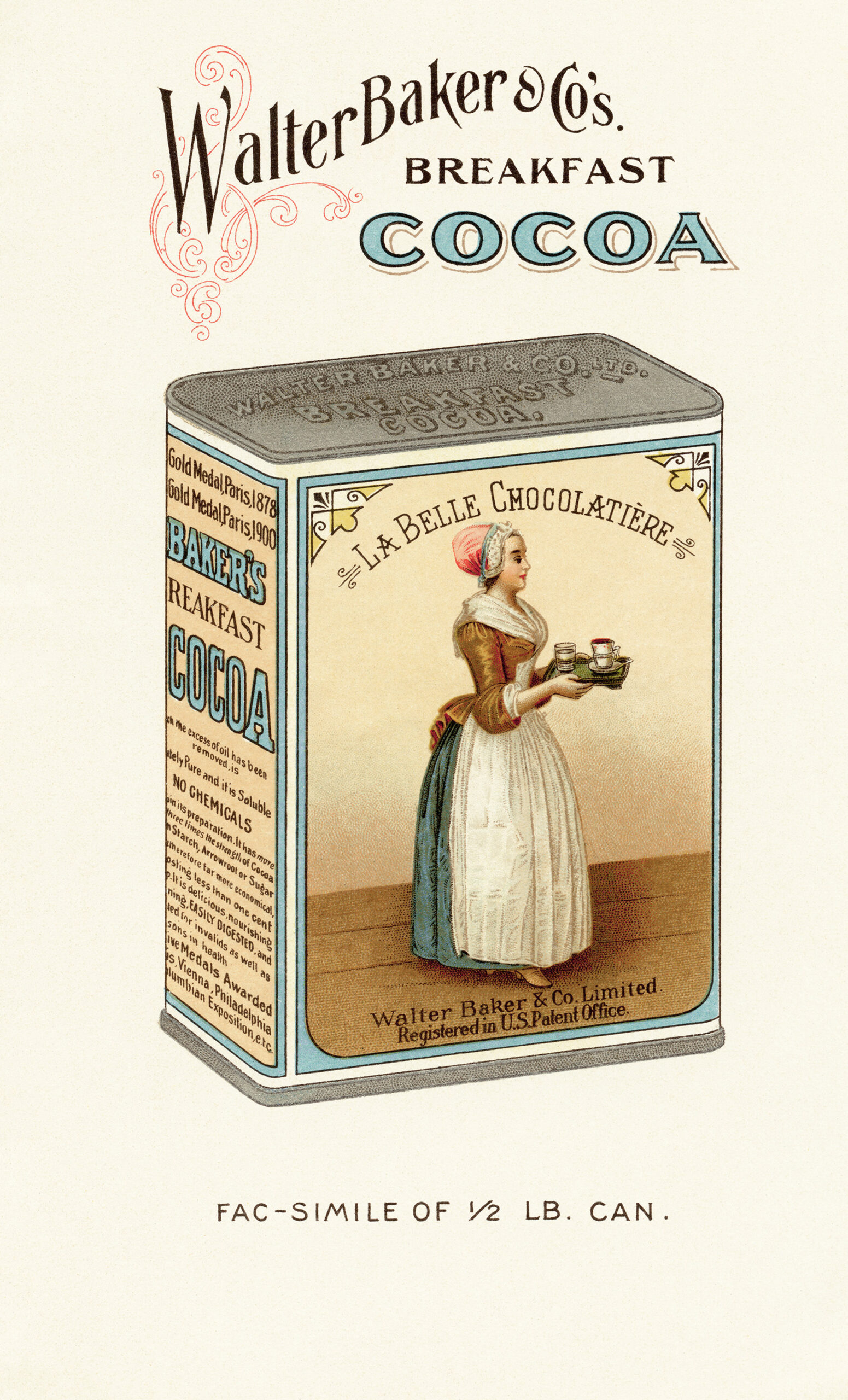This image showcases an advertisement for Walter Baker & Co.'s Breakfast Cocoa, set against a light off-white background. The main focus is a detailed drawing of a half-pound tin of breakfast cocoa, prominently labeled "La Belle Chocolatier" and featuring the text "Registered in U.S. Patent Office" on its front. The cocoa box design highlights a mid-1800s woman dressed in Victorian attire; she wears a blue and white dress, a red head bonnet, and a gold blouse layered with a white scarf. This elegantly dressed woman is depicted carrying a tray with two beverages, likely hot cocoa and another drink, possibly milk. The front side of the box features the brand name "Walter Baker & Co.'s Breakfast Cocoa" in a sophisticated black font for the company name and a thicker light blue font for "cocoa." Subtle accents in faded red embellish the "W" in Walter. Additional text on the side of the tin states "Baker's Cocoa" in blue letters and "Breakfast" in black letters, followed by claims such as "no chemicals." The background of the box is light blue, with the figure of the woman rendered in neutral shades as she stands on a brown wooden floor, adding to the vintage and charming aesthetic of the advertisement.